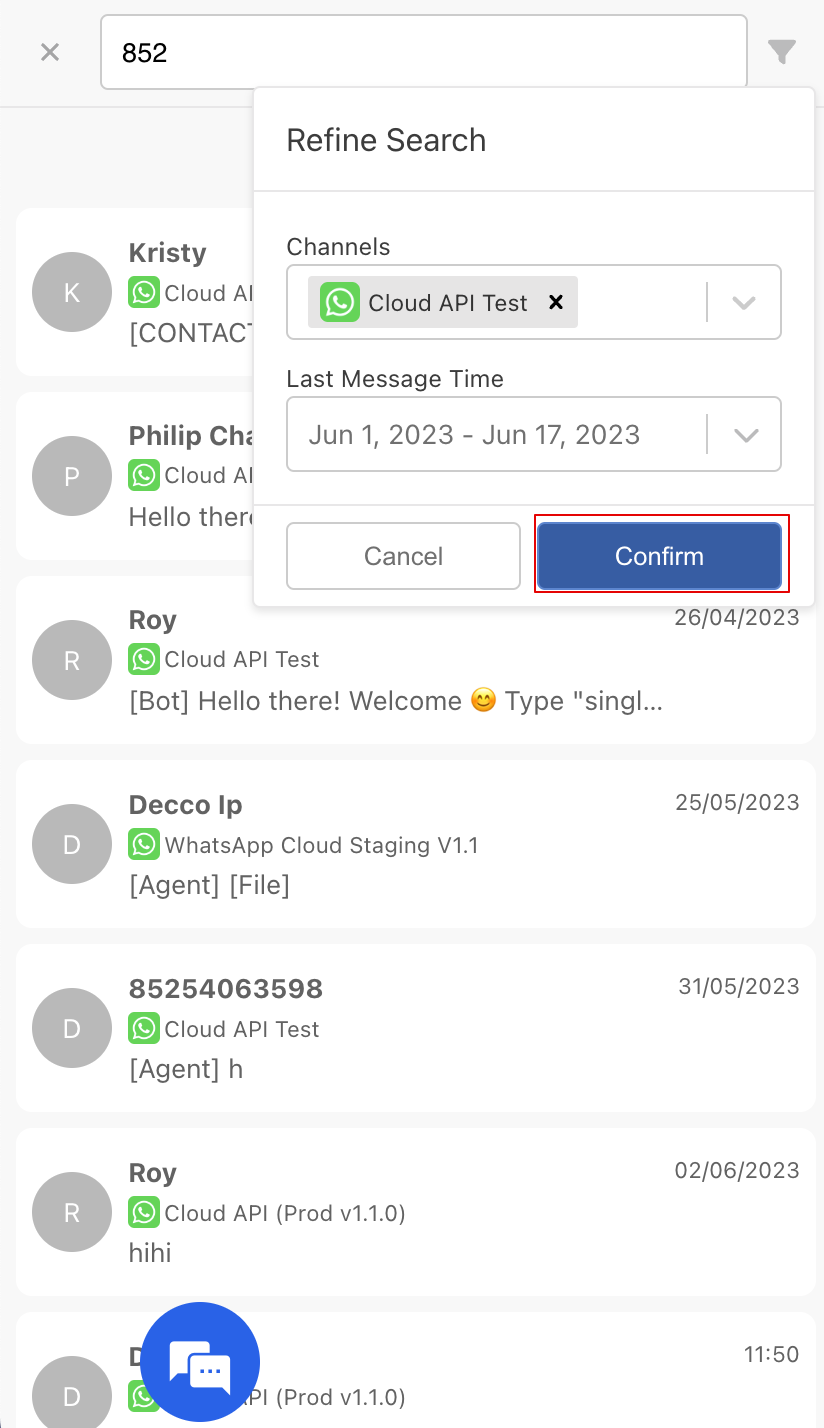This image captures a cell phone screen displaying what appears to be a messaging or contacts application, specifically WhatsApp. The background of the screen shows an interface split into distinct sections. In the top right corner, there's an additional pop-up box overlaying the main screen. 

At the very top, there is a search bar where "852" has been typed in. Below the search bar, the primary screen area reveals a list of contacts. Each contact entry features a green WhatsApp label on the left side, adjacent to a grey circle containing the first letter of the contact's name in white, capital letters.

The contact list includes names such as "Christy," "Philip," and "Roy," among others. For instance, Christy’s contact entry reads "Christy" and "Cloud API Test." Meanwhile, Philip’s entry follows a similar format, and Roy’s entry says "Hello there, welcome" beside an icon with an "R." 

There are various other entries, one of which is labeled "Deco IP" with a description mentioning it as an "agent file." Each contact is followed by relevant icons and text bubbles, respective to the messages exchanged or the status of the contacts.

At the bottom of the screen, a text bubble is present, accompanied by a refined search box. This search box provides options to "Cancel" or "Confirm" the action, with the "Confirm" button distinctly highlighted by a red rectangle and blue inner background.